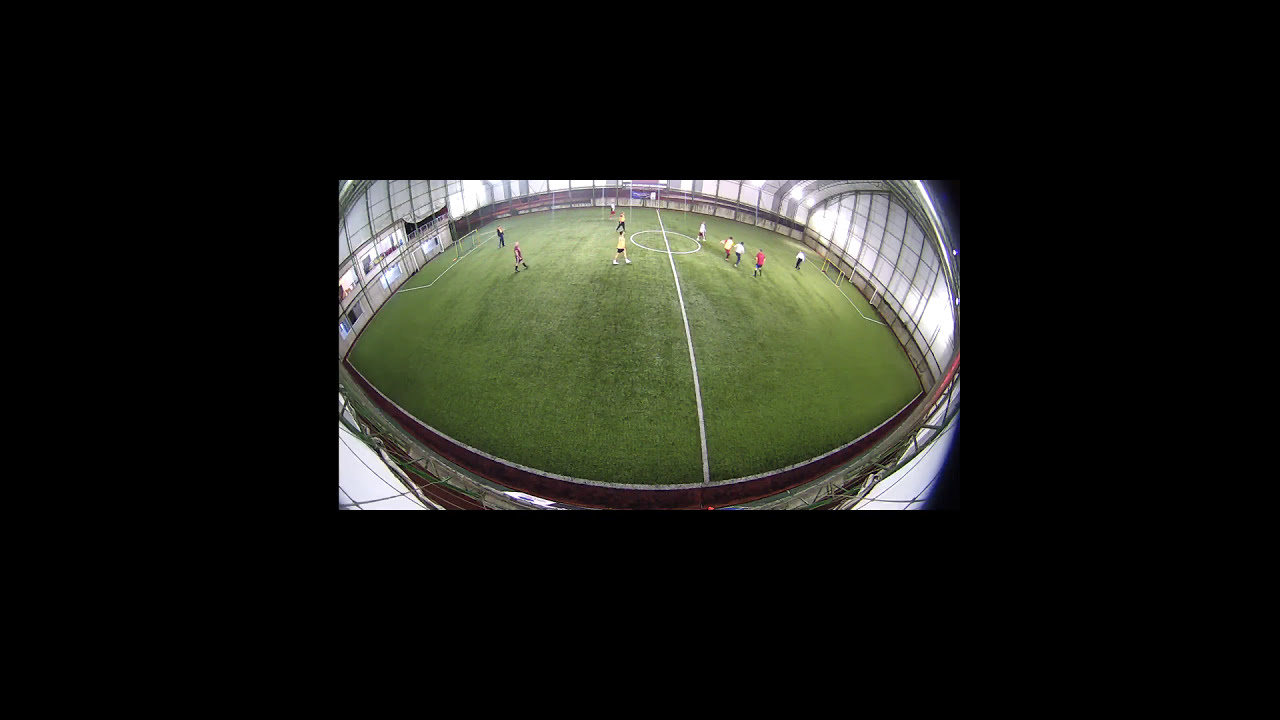This is an overhead photograph of an indoor soccer arena taken with a fisheye lens, creating a rounded-edge effect. The arena has a white dome covering with a black frame and no seating. The playing field is green and appears warped due to the lens effect, resembling a circle. A white line runs vertically through the center, intersecting with a white central circle. There are smaller goals at either end of the field, indicating a scaled-down version of soccer. The players are divided into two teams: one wearing red jerseys with blue shorts and the other in yellow jerseys with black shorts. A referee in a white shirt and black pants is also present. The arena's glass siding allows natural light to enter, particularly visible on the right side and bottom part of the photo, suggesting a retractable ceiling. The photograph captures the players in a casual stance, walking rather than actively playing, emphasizing the light, airy feel of the bright, white-dominant indoor setup.